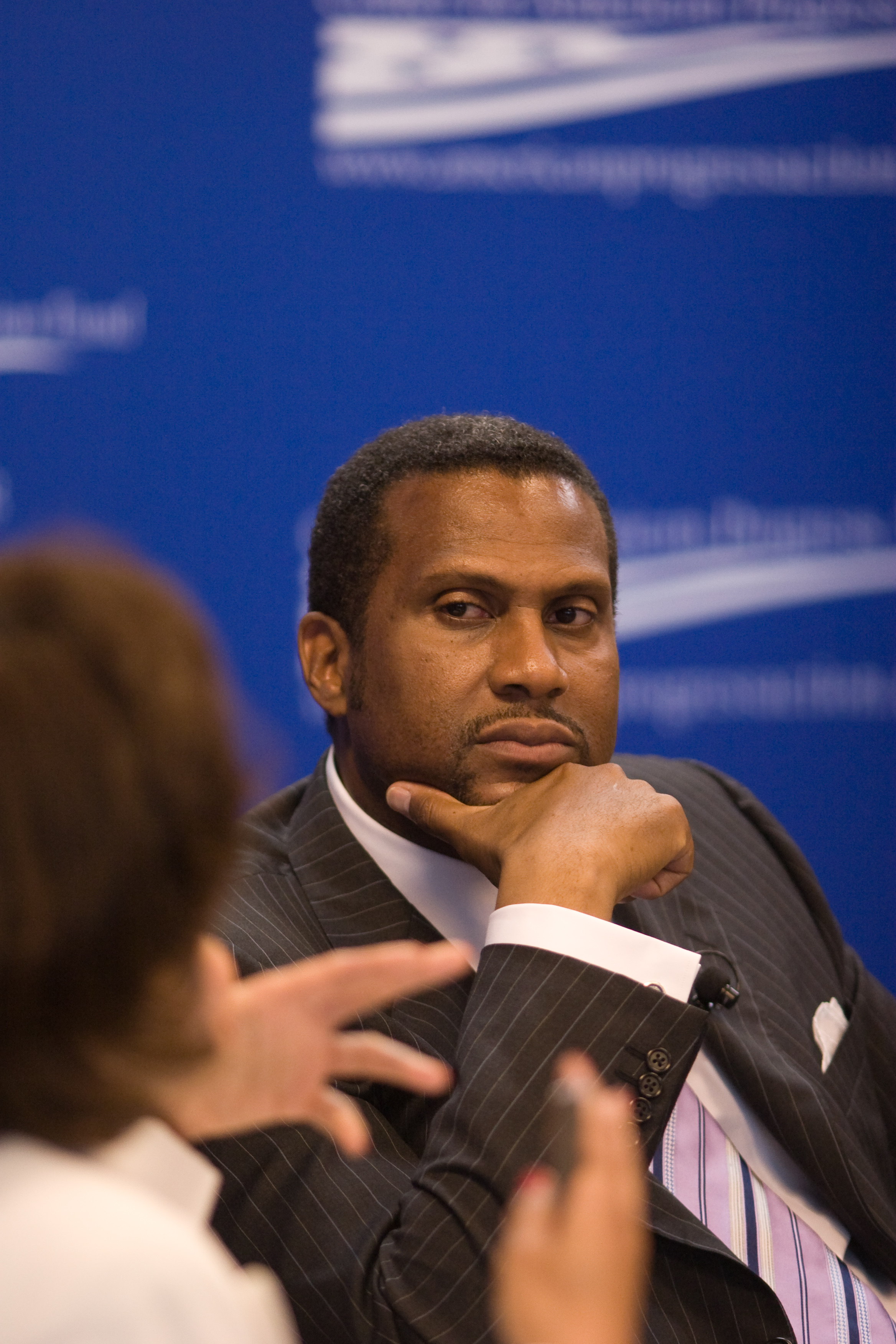The photograph captures a poised indoor scene, possibly at a press conference, with an African American man positioned centrally as the focal point. The man has short black hair and a neatly groomed mustache and goatee. He is seen sitting with his right hand touching his chin, projecting a thoughtful demeanor as he gazes intently to his left. Dressed in a dapper suit jacket with black and white pinstripes, paired with a white button-up shirt and a tie featuring shades of purple, black, and white, he emanates professionalism. 

In the foreground, to the left, the back of a woman’s head is visible, partially obscured and out of focus. She has short brown hair and is wearing a white shirt. Her hands are raised as if she is gesturing animatedly during their conversation. Behind them, the backdrop consists of a medium blue wall or signage with indistinct white logos and text, blurred beyond recognition. The color palette in the image includes hues of blue, white, brown, off-white, gray, pink, purple, and black, contrasting sharply to emphasize the subjects in the photograph.